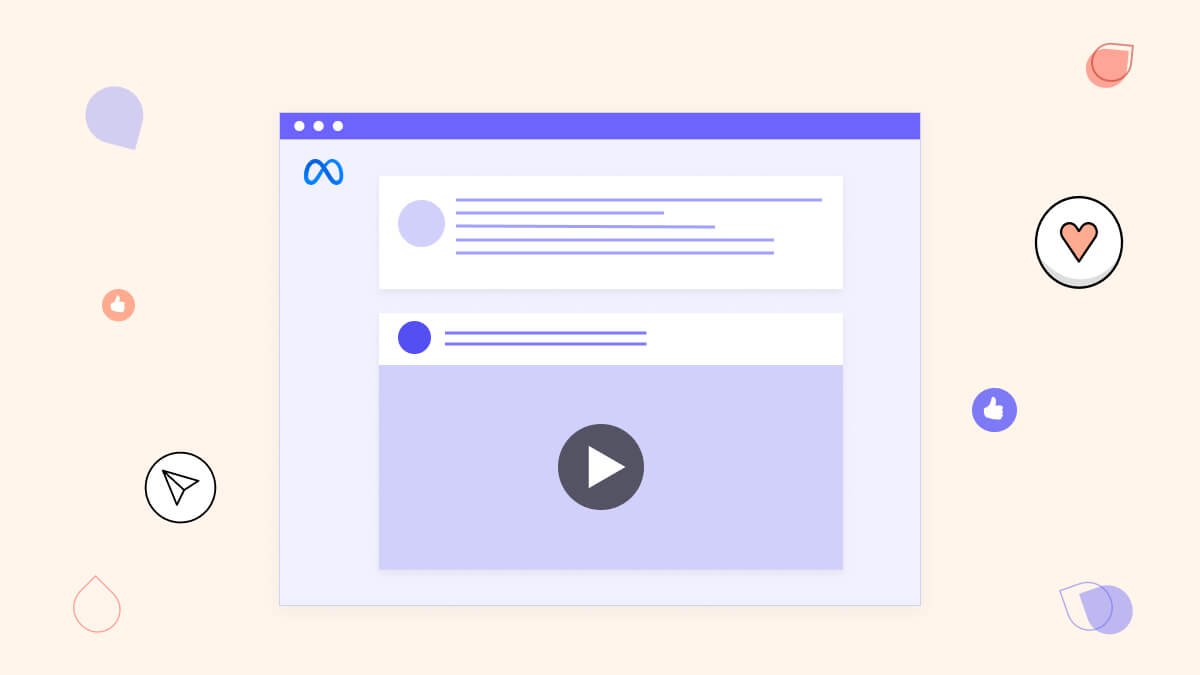This social media graphic is a large rectangular illustration with a pink background, designed to mimic an embedded view of a Facebook feed, commonly seen on the Meta app or website. In the center of the graphic, there's a prominent box showcasing an authentic-looking Facebook feed. This simulated feed features a blue top border with three white dots on the left, indicating a browser-like interface. Below the blue bar is the Meta logo on the left. Inside the feed, there are grey lines to denote where text would be in typical posts, and a second post features a play button, suggesting video content. Surrounding the central Facebook feed are various decorative shapes and social media icons. To the left and right of the graphic, hearts, thumbs up icons in pink and blue, share icons, and teardrop-shaped designs in different directions enhance the page. Additionally, there are multiple circles with embedded images: a blue circle with a pointer, a small red circle with a like hand, a white circle displaying a paper airplane, a blue thumbprint icon, a larger white circle with a pink heart, and a pink circle with a pointed end at the top. These elements collectively create a dynamic, social media-themed visual.